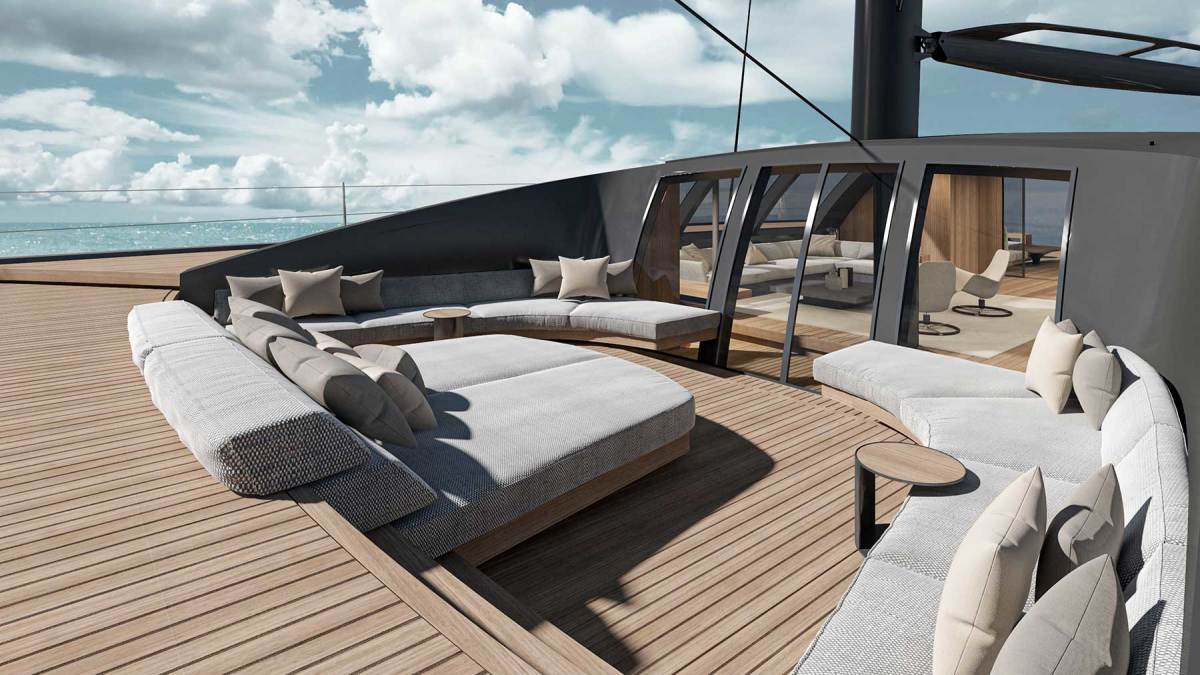The image showcases the luxurious top deck of a sleek, high-tech yacht. The deck, made from what appears to be rich mahogany wood, features several seating arrangements including a long sofa on the right with a wooden brown stool in front of it, and another similar setup on the left. Additionally, there's a larger sofa that resembles a bed, adorned with numerous pillows. 

Central to the deck is a curved sofa area with small tables ideal for socializing. Through two glass sliding doors, an inner seating area is visible, complete with a small center table and comfortable chairs. The space exudes a high-end, modern aesthetic with mirrored windows on the doors and a semi-circular wooden deck at the rear. 

In the distance, the light blue ocean and the sky with clouds provide a stunning backdrop, along with distant sailboats. The yacht also features a prominent mast, though it currently lacks a sail. The attention to detail and plush furnishings make it clear that this is a very elegant and sophisticated vessel.